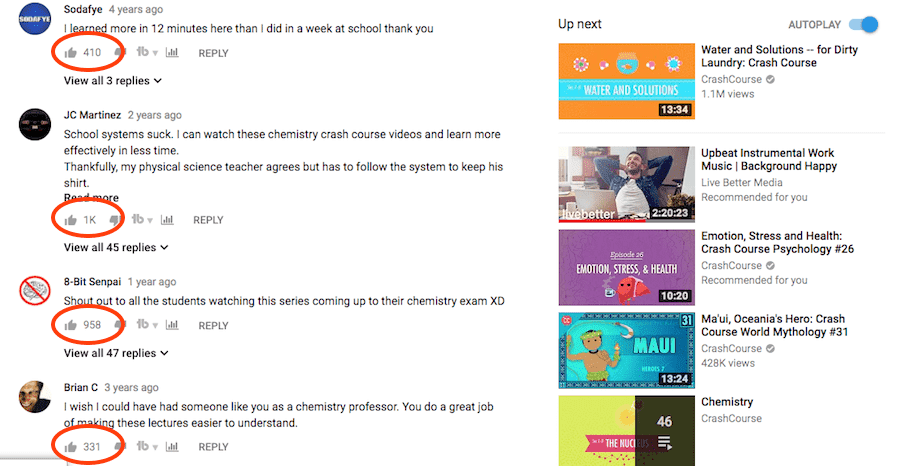This image showcases a website layout divided into two primary sections. The left section, occupying about two-thirds of the space, features user comments and testimonials. The right section hosts a series of video thumbnails.

In the comments section on the left, there is a prominent blue circle with the text "Sotify" inside it. Adjacent to this circle, it reads "Sotify FYE" and is timestamped with "four years ago." Beneath this heading, a user comment states, "I learned more in 12 minutes here than I did in a week at school. Thank you." This indicates that the section contains testimonials from students.

Further below, there's an interactive section showing a "thumbs up" and "thumbs down" icon with a count of "410" likes in between, along with an option to "view all three replies" beneath it. The three replies are displayed below, each accompanied by profile pictures on the left, with the username, time since posted, and the comment to the right. The second reply has a comment spanning four lines and shows "1K likes" with the number circled in red. The third reply consists of a single line of text with "958 likes," while the last one is a two-line comment with "331 likes."

On the right section of the page, the top left corner starts with "Up Next" in bold black text on the left side and "Autoplay" on the right. Below "Autoplay," there is a blue toggle button switched to the "on" position. Under "Up Next," there are five video thumbnails, each with a bolded black title next to the preview images. All titles comprise two lines, except for the last one, which has only one line of text. Each title is followed by a course description and its view count below.